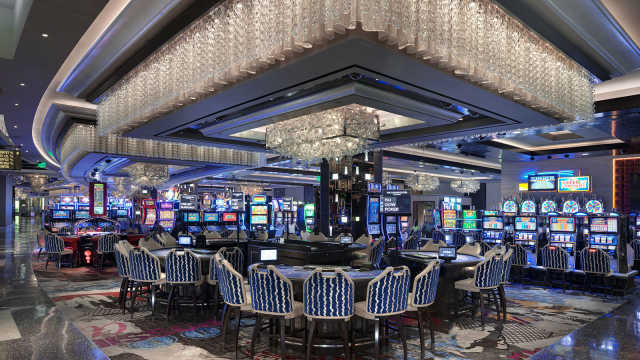The image depicts the pristine interior of a casino filled with an array of vibrant details. Centered in the photo is a section of round gaming tables adorned with blue surfaces, each surrounded by an arrangement of chairs that feature white backs with undulating patterns and black legs. Above these tables, a magnificent rectangular crystal chandelier cascades from the ceiling, bathing the scene in an opulent glow. The ceiling itself is trimmed with a ridge of shimmering white and silver crystals, enhancing the luxurious ambiance.

The casino's floor is covered with a multicolored carpet that blends hues of white, black, and green beneath the tables. In the background, long rows of slot machines are visible along the walls, each machine accompanied by a single chair – these chairs are predominantly blue but notably marked with a red square at the top of the backrest. Although the casino is devoid of patrons, the high-energy atmosphere is maintained by the lights that are fully illuminated, both on the chandeliers and the slot machines. The overall impression is one of anticipation, as if the casino is meticulously prepared and on the verge of welcoming its next wave of guests.